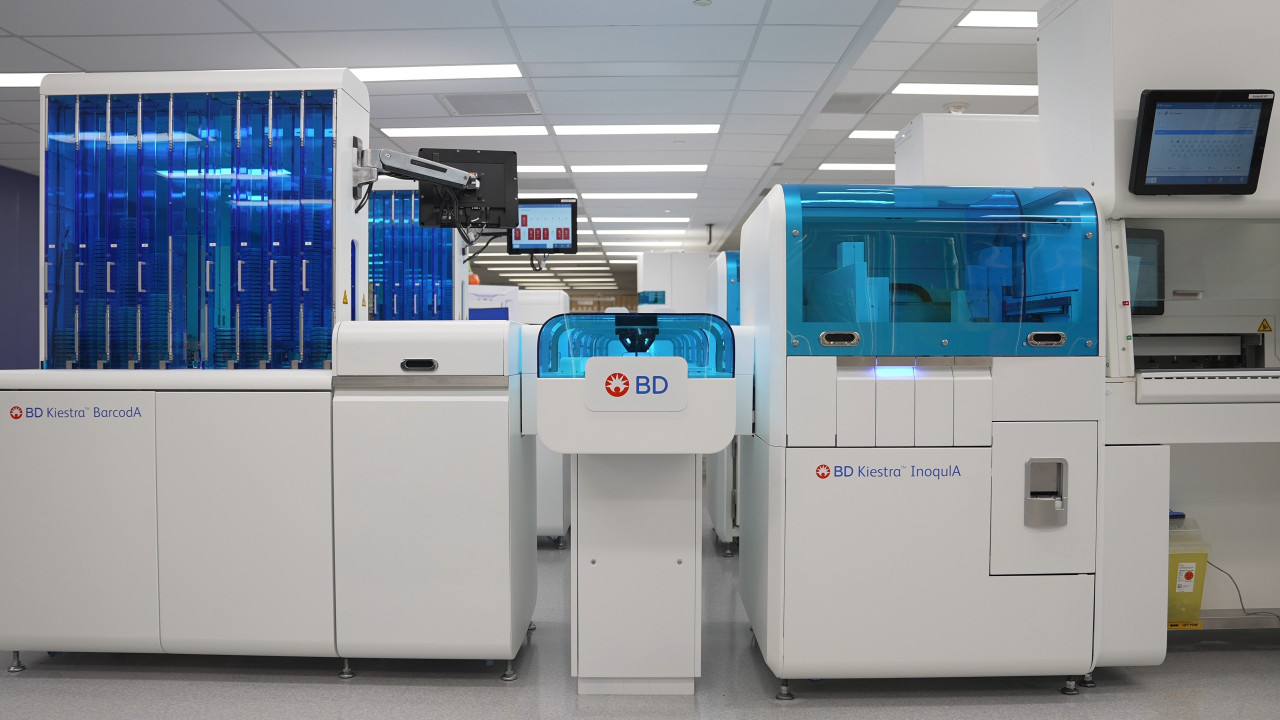The image depicts a meticulously clean and modern office space, potentially within a hospital or a high-tech factory setting. The office is furnished with smooth gray flooring and a ceiling lined with white tiles, some of which have integrated lights designed to blend seamlessly with the tiles. The room houses several white, bulky machines with rounded corners, all bearing the brand name "BD Kiestra Inaquia," a few models being labeled as "Kiestra Barcodea" and "Kiestra Inaquia."

The largest machine, positioned on the left side of the image, features a clear blue transparent section that hints at the intricate technology inside without fully disclosing its purpose. Adjacent to it is a slightly smaller machine with a less prominent, yet similarly blue-hued, see-through component. The smallest and thinnest machine sits in the middle, standing at about three feet tall. To the right, a larger machine about four feet tall and three feet wide completes the primary foreground trio.

Scattered around these machines are computer monitors, suggesting a space where scientific or technical analysis occurs. The room's pristine condition, with reflective flooring and a new appearance, enhances its professional and high-tech ambiance. Blue-tinted windows add a touch of color and natural light to the otherwise sleek white and gray interior, reinforcing the impression of a cutting-edge workplace.